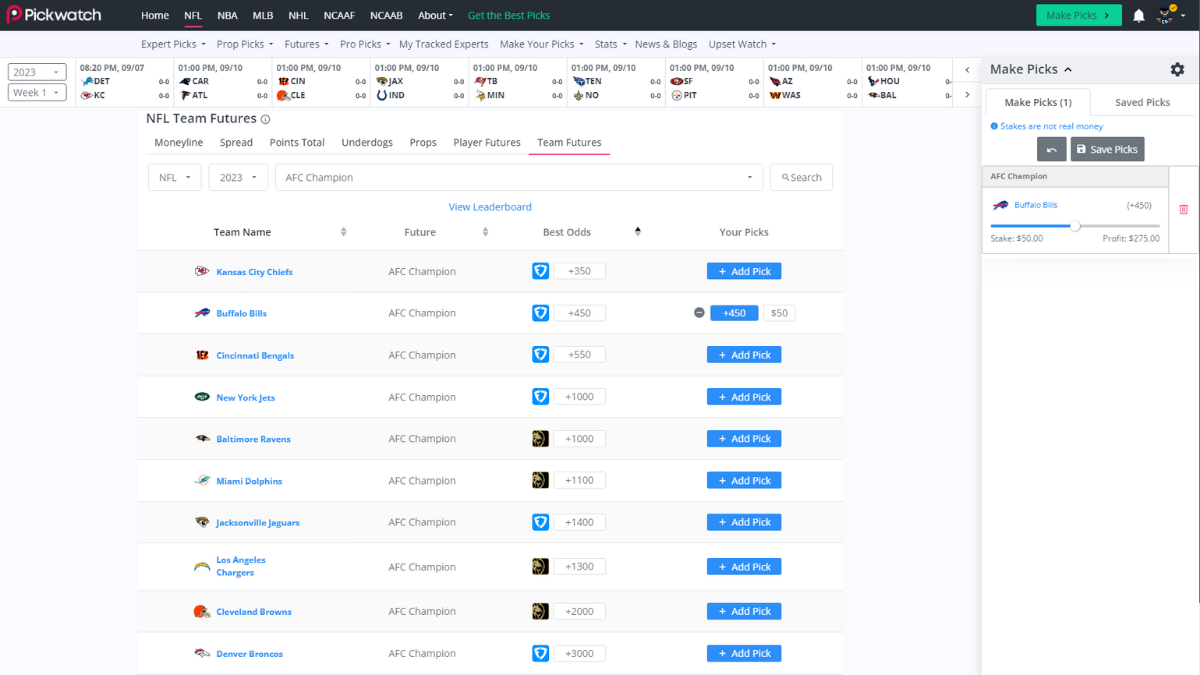This image captures a detailed screenshot of the Pickwatch sports betting application, presented in a landscape orientation. The background is predominantly gray, while the top edge is marked by a horizontal black border. On the left side of this border, there is a distinctive "P" icon outlined in red with a white dot at the center, accompanied by the word "Pickwatch" in white text.

Within the black border, the app interface includes a horizontal navigation bar with several options. From left to right, the options are: Home, NFL, NBA, MLB, NHL, NFL (again), and College Basketball. Currently, the NFL option is selected, indicated by a red underline. Adjacent to these options, there is a green text prompt that says "Get the Best Picks," followed by a green box labeled "Make Picks" and an icon for notifications.

Below the navigation bar, the app displays an NFL schedule section with drop-down boxes, where "2023 Week One" is currently selected. The main content area of the interface shows betting options, with "Team Futures" highlighted by a red line. The screen provides a list of NFL teams along with their odds for becoming the AFC Champion. At the top of this list are the Kansas City Chiefs, with options for placing bets through platforms like FanDuel and MGM. Additionally, there is an option to add a pick.